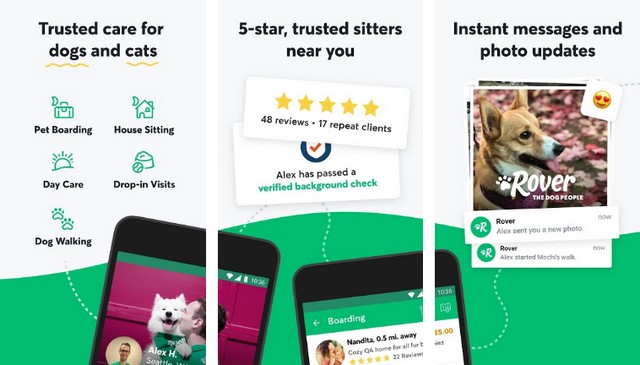The image consists of three distinct rectangles that together form a cohesive scene. The overall design is in a flowing wave shape, transitioning from white at the top to green at the bottom. 

**Left Rectangle:**
- Contains the text "Trusted care for dogs and cats" in black font. The words "dogs and cats" are underlined with a gold squiggly line.
- Below the text, there are icons with labels indicating various pet services: Pet Boarding, House Sitting, Daycare, Drop-in Visits, and Dog Walking.
- Includes an image of someone hugging a fluffy white dog against a purple background, spread across this and the middle rectangle.

**Middle Rectangle:**
- Features the text "Five-star trusted sitters near you" along with a five-star review rating, 48 reviews, and a note that 17 clients are repeat customers. 
- Highlights that "Alex has passed a verified background check."
- Shows a phone image that straddles the middle and left rectangles, listing other potential sitters and their ratings.

**Right Rectangle:**
- Promotes "Instant messaging and photo updates" with a picture of a dog named Rover, including a heart-eyed emoji icon.
- Displays various pictures of Rover.

Each rectangle is thoughtfully integrated, creating a unified visual that communicates trust and comprehensive pet care services.